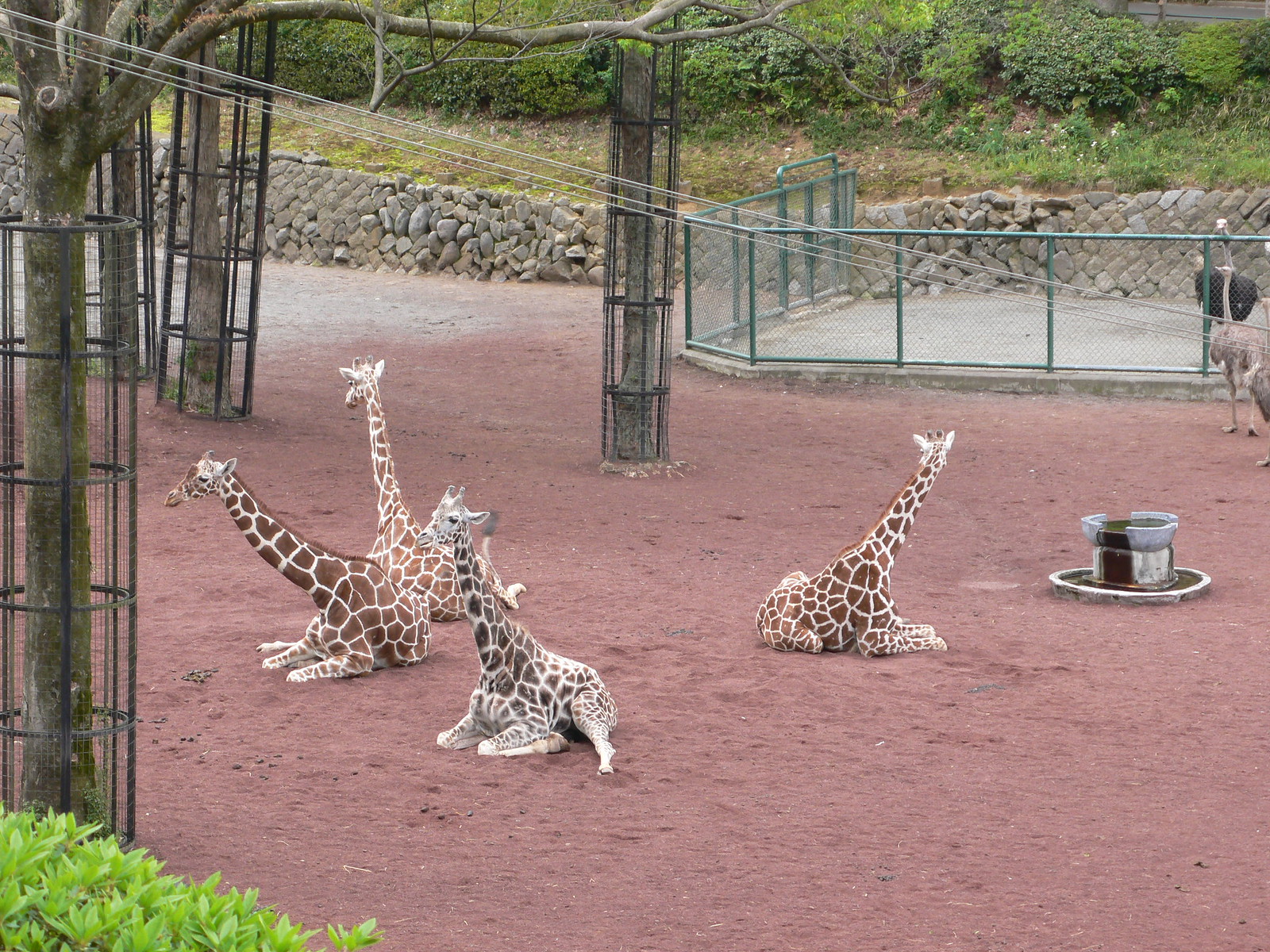In this landscape-oriented color photograph taken at a zoo, we see a group of four giraffes sitting on reddish, clay-like dirt ground, with impressions indicating its soft texture. All giraffes have their legs tucked under their bodies, except for one in the foreground, which has one back leg stretched out in front. To the back and right, within the same enclosure, there are several ostriches: one with lighter tan feathers slightly cut off from the screen, and another darker-feathered one near the chain-link fence. The background reveals green fencing with a stone wall made of differently shaded gray bricks, above which is a grassy hedge and bushes. Further left, three tall trees are protected by cages made of bars and mesh to prevent the animals from damaging them. The edges of the image feature green shrubs, with some light green foliage in the foreground, hinting at the photographer’s elevated viewpoint from a likely viewing platform.